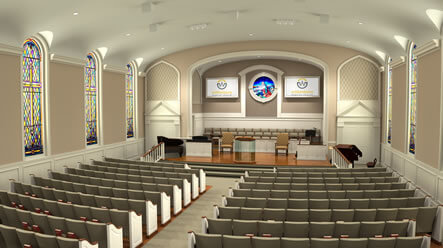The image depicts the interior of a small church, characterized by a serene and inviting atmosphere. The church features rows of individual, auditorium-style seating with dark brown fabric cushions for congregants, with aisle walkways dividing the seating sections on either side. The end of each pew is highlighted by white coloring. 

The church’s walls are painted a neutral beige tone, contrasting against the white ceiling, and are adorned with colorful, large, tall stained glass windows on both sides. Each side of the church has three stained glass windows, which sport a rainbow collection of colors and share a consistent design. 

At the front of the church, a prominent wooden stage is seen, flanked by gray steps. At the center of this stage, under a smaller arch, is a circular stained glass window, adding an element of classical ecclesiastical architecture. Above the stage, two rectangular screens are mounted on either side of the circular window. Below the screens, there are additional rectangular boxes with writing and imagery that are hard to discern from the distance. 

The stage accommodates several elements, including a piano on one side, large brown chairs, and additional chairs likely intended for choir members or speakers. The presence of Bibles sticking out from the back of the seating and the overall emptiness suggest that the image was taken in a quiet moment, possibly before a sermon or gathering. 

Together, the white rails leading up to the platform, the light gray-colored carpet, and the wooden elements on the floor stage area complete the harmonious and contemplative setting of this church interior.